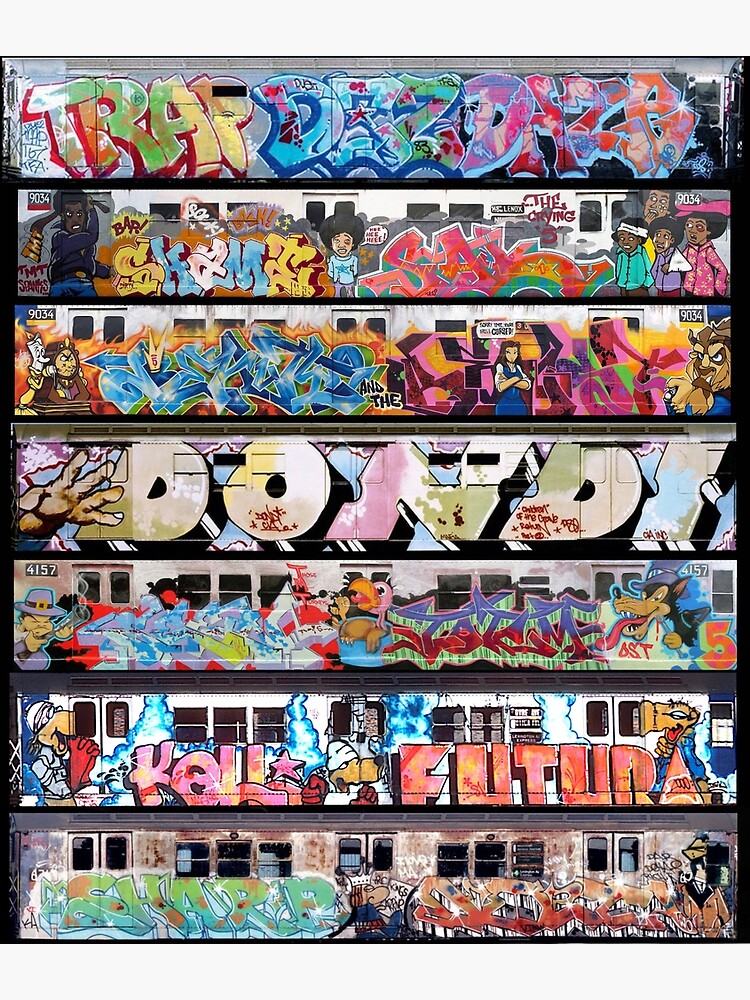The image showcases a vibrant collage of street art graffiti, likely from an abandoned high-rise in downtown Los Angeles, detailed across seven distinct rows. The graffiti adorns what appear to be either buses or trains, with doors, windows, and number markings visible through the artworks. Each piece is a colorful display of professional artistry featuring multicolored letters, intricate designs, and evocative imagery. Notable pieces include: a name emblazoned in rainbow colors with stars and colorful splotches, a depiction of people with one character's quote bubble highlighted, and a detailed "Beauty and the Beast" scene with familiar characters like Belle, the Beast, the clock, and the candlestick. Some tags include the names "traps," "shams," and "dandy," while others show a mix of blues, purples, and darker shades. The caption “Cole Futura” is notable in white and red lettering against a clean backdrop. Overall, this vivid collection transforms the urban landscape into a dynamic and colorful museum of street art.